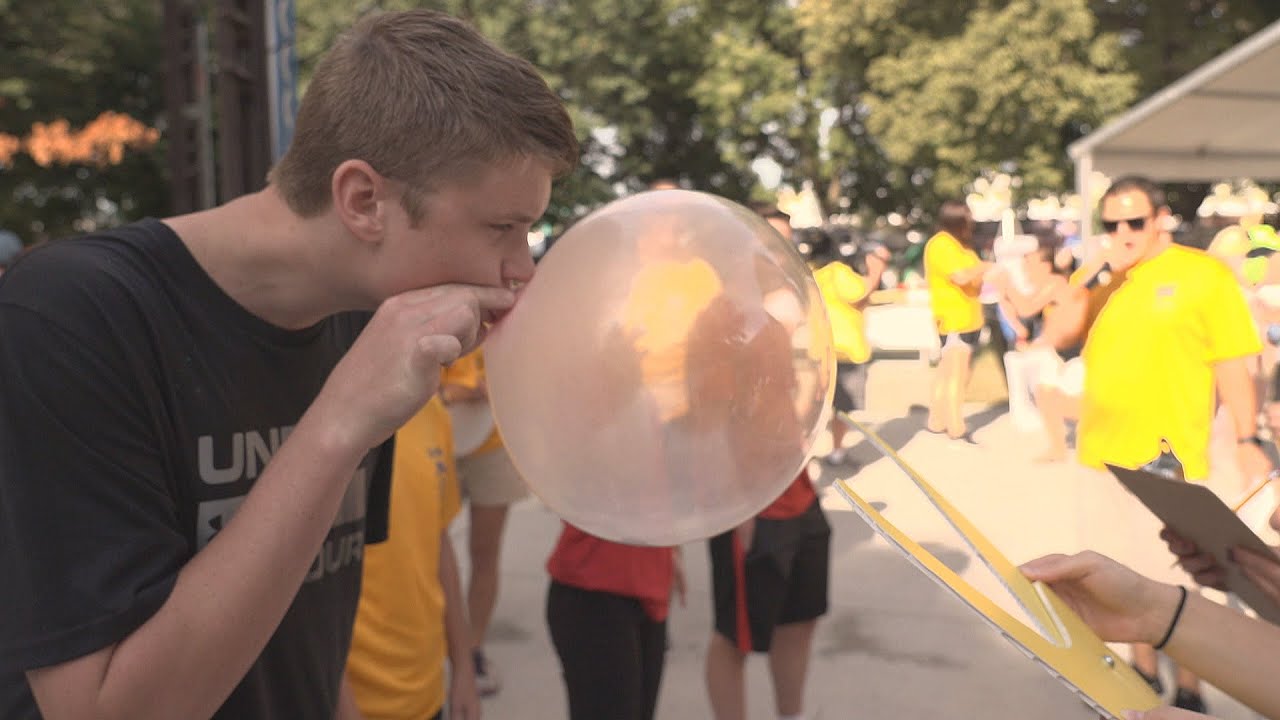In this photograph, a lively gathering is taking place, featuring individuals predominantly dressed in yellow or orange shirts, blurred in the background among trees and a small shelter, creating a vibrant setting. Dominating the scene is a young man with short brown hair, dressed in a black t-shirt, who is the focal point as he blows up what seems to be either a balloon or a bubble from a piece of gum, positioned in the center of the photo. To the right of the bubble, a pair of hands holds what appears to be a measuring tool, possibly to determine the bubble's circumference. In the background, specifically on the right, stands a gentleman in a yellow t-shirt and sunglasses who is observing the scene. Behind the bubble, two individuals in red shirts—one with black pants and the other with a hand in their shorts pocket—are visible, contributing to the social ambiance of the gathering.